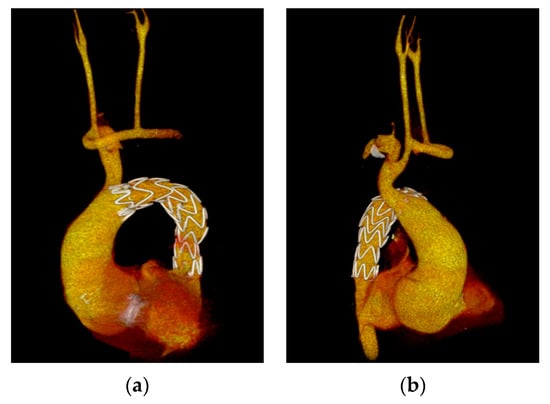The image consists of two side-by-side pictures labeled "A" and "B," showing what appears to be the same yellow object with a black background. The object, difficult to identify precisely, resembles an abstract or artistic representation of an animal or a crafted figure. It has a circular lower body with thin upper extensions that could be branches or legs. The circular part of the body features white zigzag patterns, possibly resembling thread or frosting, and the bottom has a reddish, fuzzy appearance. The inconsistency in identifying whether it's falling or simply positioned against the black makes the interpretation challenging, but the vivid use of yellow, black, white, and red adds to its enigmatic presence.